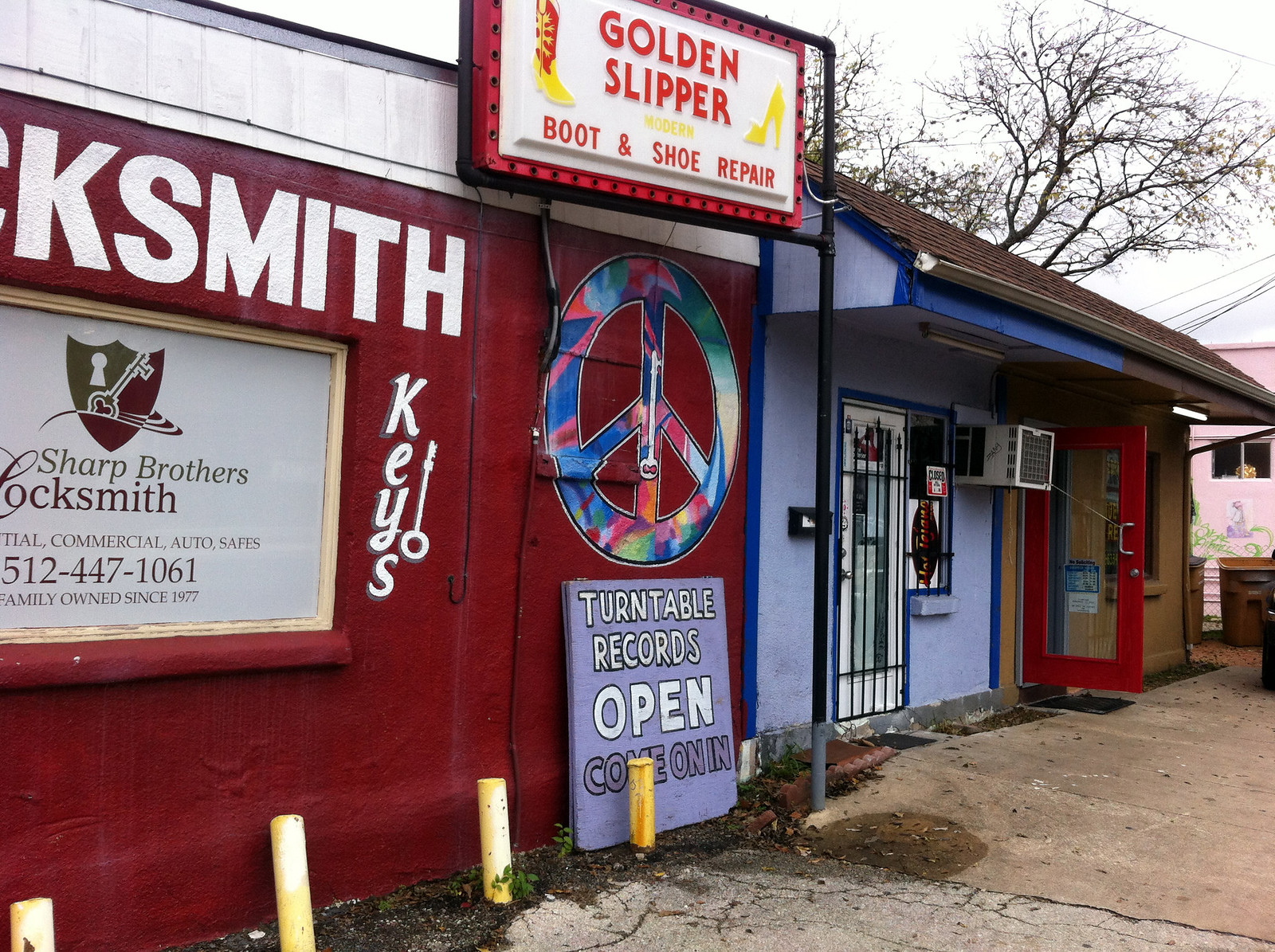The image captures a quaint, single-story storefront that houses multiple businesses. Dominating the left side is a section with a red background bearing the name "KSMITH" in bold white capital letters. Below this, the sign reads "Sharp Brothers Locksmith, Residential Commercial Auto Safes," along with a phone number, "512-447-1061," and the note, "family owned since 1977." Adjacent to this is a smaller sign advertising "Keys."

In the center of the storefront, another prominent sign announces "Golden Slipper Boot and Shoe Repair." Below this sign is a large, tie-dyed peace symbol. Further down, another sign invites patrons to "Turntable Records Open, Come on in."

To the right, a blue-painted building features a gated front door with an air conditioner jutting out above it. Nearby, an open door with a red outline is held ajar by a bungee cord. In the background on the far right, a pink building can be seen. The area around the storefront is characterized by cracked pavement and the scene is set outdoors with a large tree and a white sky visible above.